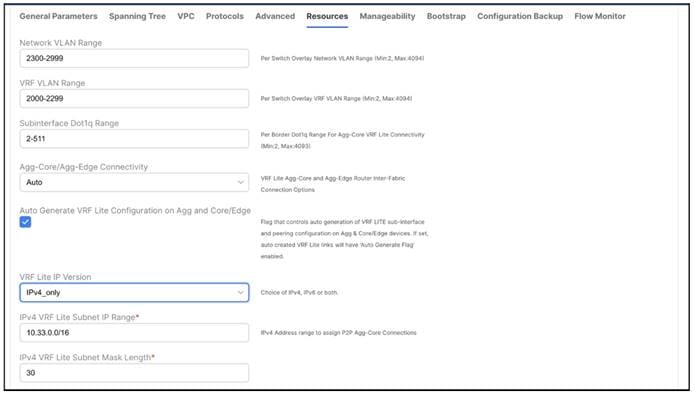The image depicts a detailed configuration page from a network management interface. The white background features black text categorized under various headers:

1. **General Parameters:** 
   - Spanning Tree
   - VPC (Virtual Port Channel)
   - Protocols
   - Advanced Resources

   A blue underline separates this section from the next.

2. **Manageability:** 
   - Bootstrap
   - Configuration Backup
   - Flow Monitor

3. **VLAN Range Management:**
   - VLAN Range 2300-2999 (for Network)
   - VRF (Virtual Routing and Forwarding) VLAN Range 2000-2299
   - Subterranean Doral Range 2-511

4. **Connectivity Settings:**
   - Aggregate Core (Ag Core) and Aggregation (Aggage) Auto Connectivity
   - Auto-Generate VRF Lit Configuration on Aggregate and Core

5. **VRF Lit Settings:**
   - VRF Lit IP Version set to IPv4 Only
   - VRF Lit Submit IP Ring: 10.33.0.0/16
   - VRF Lit Submit Mask Length: 30

The overall configuration page is meticulously organized, with each setting clearly labeled and spaced for ease of navigation.